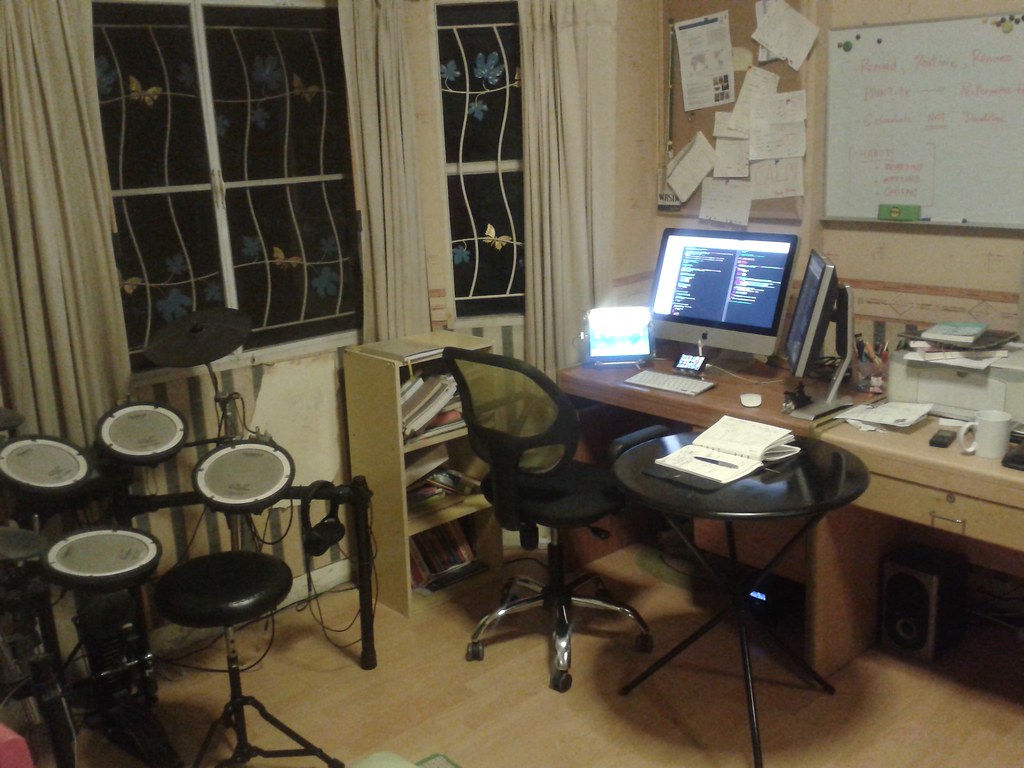This photograph captures a cluttered and multifunctional office space within a home, serving as an office, hobby room, and music studio. The right side of the image features a light wooden desk topped with a dual Apple monitor setup displaying coding text, a small tablet, a lit telephone, and a white coffee cup. In front of the monitors, there's a tiny white keyboard and a computer mouse. The desk is adorned with a plethora of papers and miscellaneous items, and a white printer stacked with various objects sits to the right. Above the desk are a whiteboard with red writing, blurred but legible, and a bulletin board densely pinned with papers and post-it notes. 

A modern ergonomic black swivel chair with mesh back and reflective silver leg supports sits in front of the desk. Adjacent to the chair on the right is a small round black table with three legs, holding an open notebook with a pen and remote control. To the wall’s left resides a small three-shelf bookcase filled with books and assorted items, positioned in front of two large windows. The windows have light-filtering white curtains drawn open to reveal metal bars forming a distinctive wavy pattern.

The room's floor is light yellow hardwood, and its beige and olive green striped wallpaper contrasts with the white elements scattered throughout. On the room’s left side, an electronic drum kit complete with a stool and cymbal suggests a musical element to the room's purpose. The atmosphere is further characterized by its somewhat cluttered arrangement and dimly lit, night-like ambiance outside the windows.